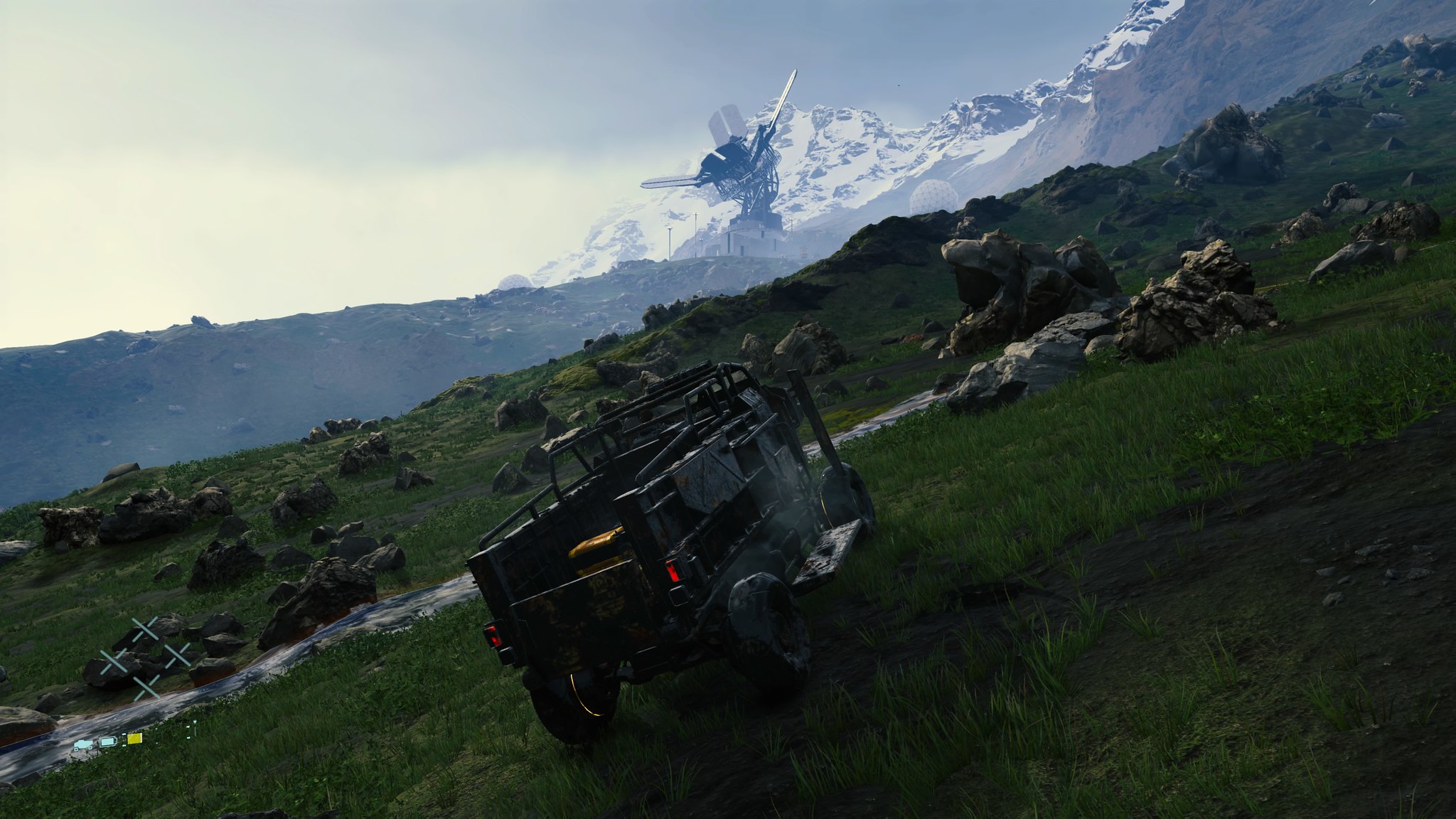This image, likely from a high-resolution video game, depicts an expansive, hilly landscape lush with green grass interspersed with darker patches of dirt or mud. Prominent rock outcroppings and boulders are scattered across the grassy plain. In the foreground, a dark green or gray army jeep-like truck is visible, featuring an open cab and cargo in its flatbed. The vehicle has functional elements, including two lights and a yellow detail on its back. A notable HUD (heads-up display) overlay appears in the lower-left corner, adorned with a logo of four white Xs and small colored symbols.

In the distance, a massive, snow-capped mountain range stretches across the background underneath a light blue-gray sky, which fades to almost white on the left side. Atop the highest peak, a futuristic-looking satellite dish or signal booster stands, its structure partly opened, resembling the equipment from a high-tech outpost. Smaller mountains form a secondary horizon line below the major peaks, adding depth to the scene. The weather is a mix of clear skies and puffy white clouds, imbuing the image with a serene yet slightly overcast atmosphere. Among the details in the image, small creatures or robots can be vaguely made out against the hilly terrain, enriching the game landscape's immersive quality.